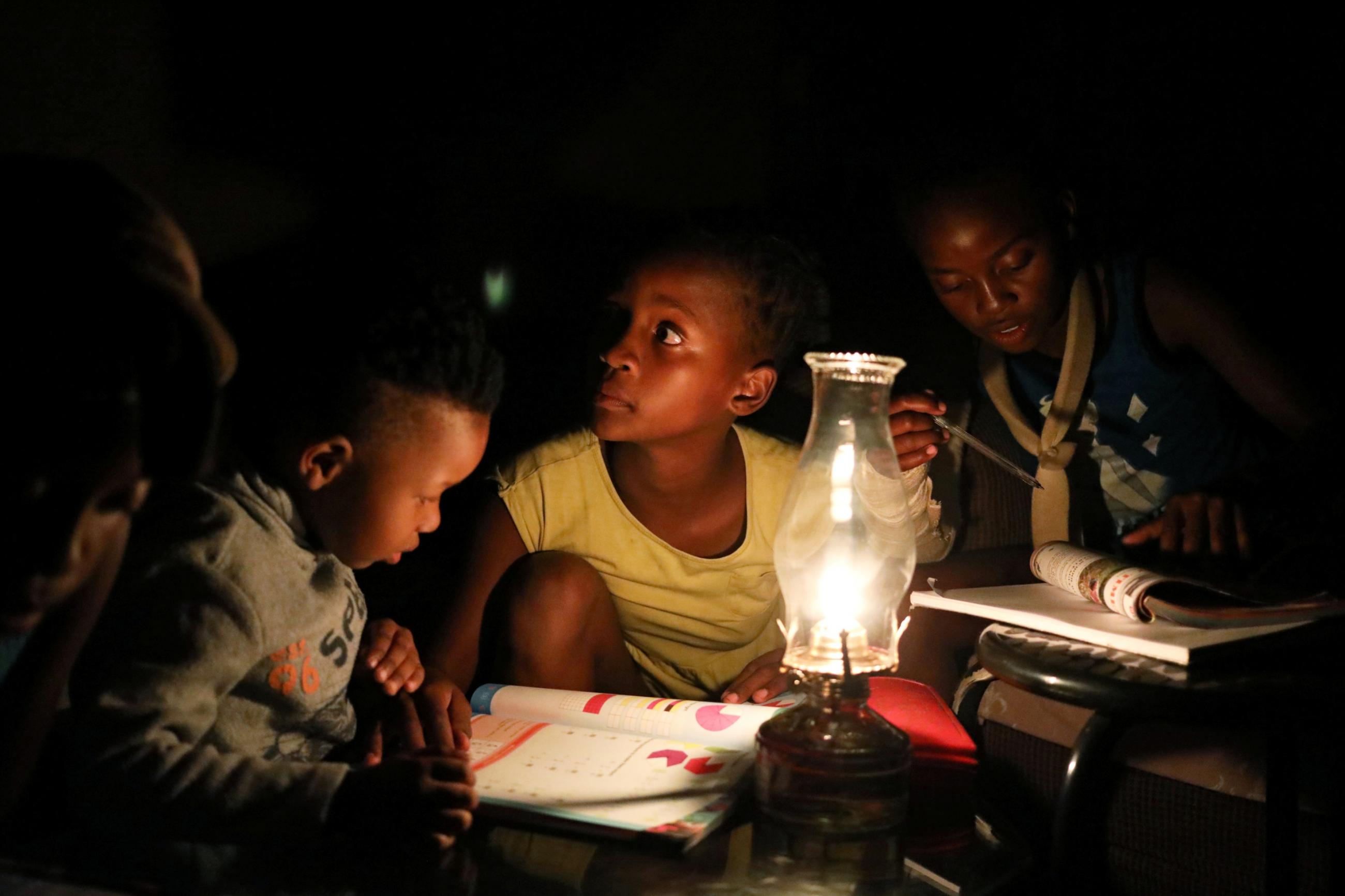The image captures three black children of varying ages engaged in a paper-based activity against a pitch-dark background, with only a green light faintly glowing in the distance. The scene is illuminated by an old hurricane lamp placed on a wooden table, casting a warm glow over the group. The youngest boy, positioned at the left, with short black hair and wearing a gray sweatshirt, intently studies the middle boy's math homework. The boy in the middle, seemingly older and dressed in a yellow shirt, gazes towards the left, possibly observing something out of frame. Across from him sits a girl in a light green short-sleeved t-shirt, her left hand gently clutching the lamp. She too is looking upward towards the left. This intricate composition is anchored by their focused expressions and the solitary lamp, establishing a serene yet studious atmosphere.